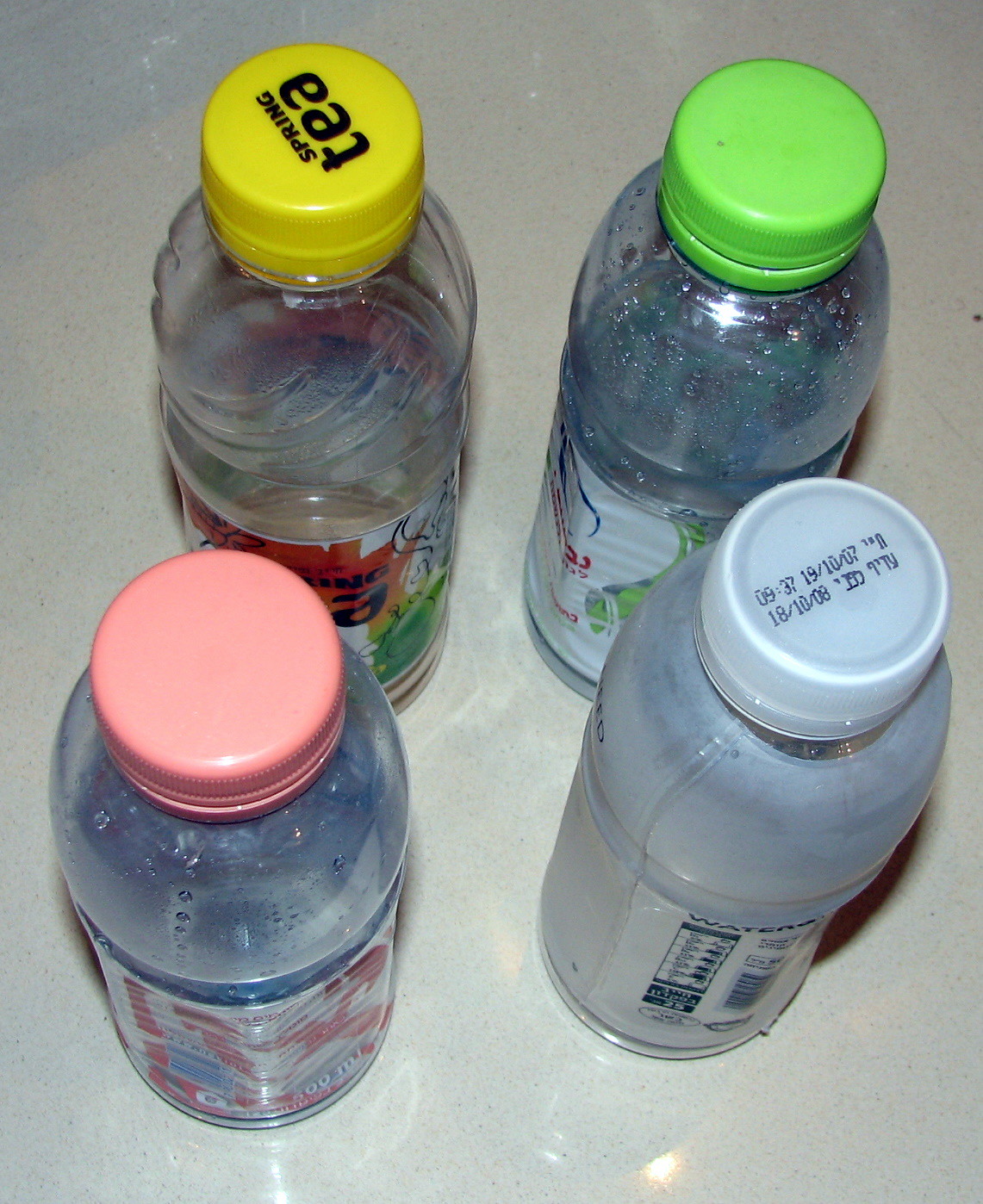The image features four distinct plastic drink bottles placed on a shiny, white speckled surface, likely a table. Each bottle has a different colored lid and label, adding to their unique appearances. Starting from the top left, there is a bottle with a yellow lid labeled "Spring Tea," featuring a red, green, and white design, visibly containing some dark liquid at the bottom. Next, on the top right, is a bottle with a bright highlighter-green lid and a mostly white label, though the exact contents are unclear. Moving to the bottom left, there is a bottle with a pale peach lid adorned with a label that includes both white and pink colors. Finally, the bottle on the bottom right has a white cap with numerical details, labeled as water. All the bottles appear to be largely empty, with only slight traces of liquid residue remaining. The perspective of the image is from a top angle, showing more of the bottle lids and some details of the front but making the labels somewhat difficult to read. The variety in design and potential non-English text hints that these bottles could be from an international origin, perhaps Japan or Korea.